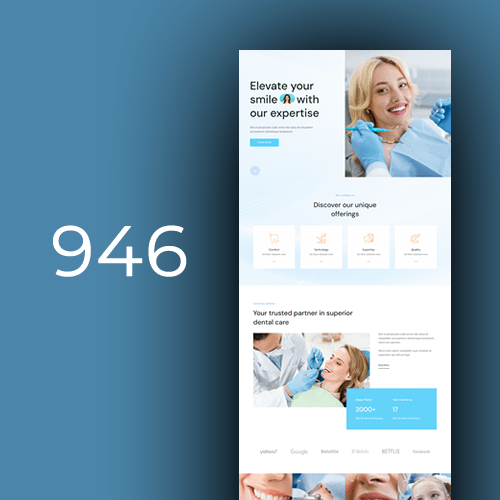The image appears to be an advertisement likely intended for a magazine, website, or banner ad. 

The background is a vibrant teal blue. On the left side, the background remains solid teal blue, featuring the bold, white number "946" prominently in the center.

The right side of the image contains various elements on a white vertical rectangle:

- At the top, the phrase "Elevate your smile" is written in black, accompanied by a small blue cartoon icon of a woman.
- Following this is a line of small black text that is indistinguishable followed by a turquoise rectangular bar with white, unreadable lettering.
- In the upper right corner, there is a picture of a woman sitting in a dentist's chair, smiling, with a blue napkin around her neck. A dentist's gloved left hand holding a dental pick is visible. 
- Beneath this image is a line of small blue text that is also too small to read.
- The text "Discover our unique offerings" is written in black below this image, with four horizontally aligned white squares beneath it. Each square contains an orange-yellow icon and a line of black text that is too small to read.
- Below these squares, the phrase "Your trusted partner in superior dental care" is written in black. Adjacent to this, there is another imagery— a woman undergoing a dental procedure with the dentist's head and hands visible.
- To the right, small unreadable black text appears just below this image.
- Beneath, a blue rectangle features the numbers "2000" and "17" in white against more white lettering that is too small to read.
- At the bottom of the white section, a series of black, horizontal labels are again too small to decipher.
- Along the bottom edge, there are four small photos of smiling mouths.

The advertisement effectively introduces viewers to an emphasis on quality dental care, although many text details are too minute to be read clearly.